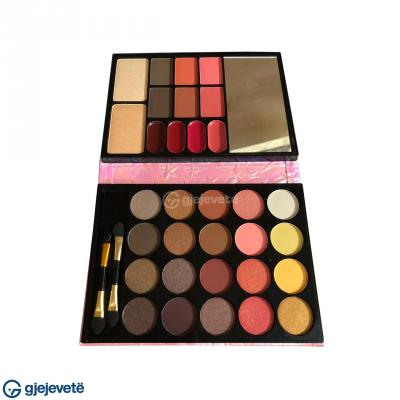This image features a two-piece makeup palette designed for eyeshadow application. The lower half of the palette displays a case that opens up to reveal 20 circular eyeshadow colors arranged in four rows and five columns. These colors range from vibrant hues like bright yellow, green, blue, pink, and red, to deeper shades including dark red and brown. Two signature silver eyeshadow applicators rest on the left side in a dedicated tray. 

Separating the two sections is a pinkish strip, likely serving as a hinge when the palette is closed. The top half of the palette includes a large mirror on the right side, extending from the top to the bottom of the packaging. This section contains a variety of eyeshadow colors in six square pans, four capsule-shaped pans, and two long rectangular pans. The colors here span various tones of reds, with several pale shades on the left. Additionally, in the bottom left corner of the palette, there is a circle containing the letters "G-Y-E-J-E-B-E-T-E."

Together, these elements create a comprehensive and versatile eyeshadow palette, providing a wide spectrum of colors for different makeup looks, with mirror and brushes included for convenient application.